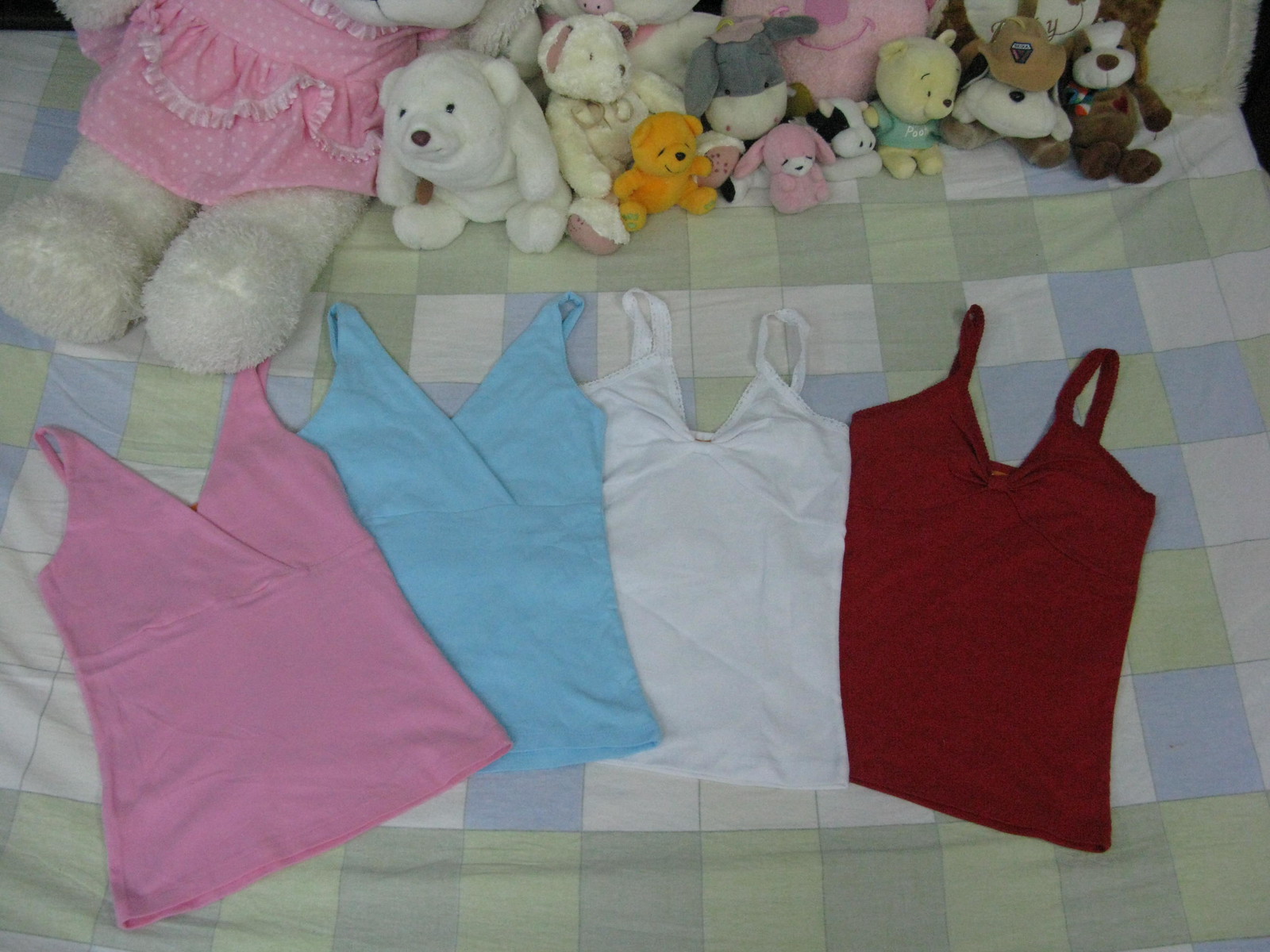This image captures a detailed arrangement on a neatly made bed with a checkered comforter featuring squares in light blue, green-blue, and white. On top of the bed, four spaghetti strap tops for women, all of the same size and style, are meticulously laid out side by side. From left to right, the tops are pink, baby blue, white, and red. Above these tops, a diverse collection of stuffed animals is displayed, spanning from the top left to the top right of the image. The plush toys include various animals such as bears, rabbits, a dog, a polar bear, a donkey, a cow, and a distinct yellow bear resembling Winnie the Pooh with a green shirt. There's also a larger stuffed animal in a pink dress and one with a pink happy face. These stuffed animals are arranged upright against pillows, suggesting a cozy, personal space, possibly a child's or a teen's bedroom.